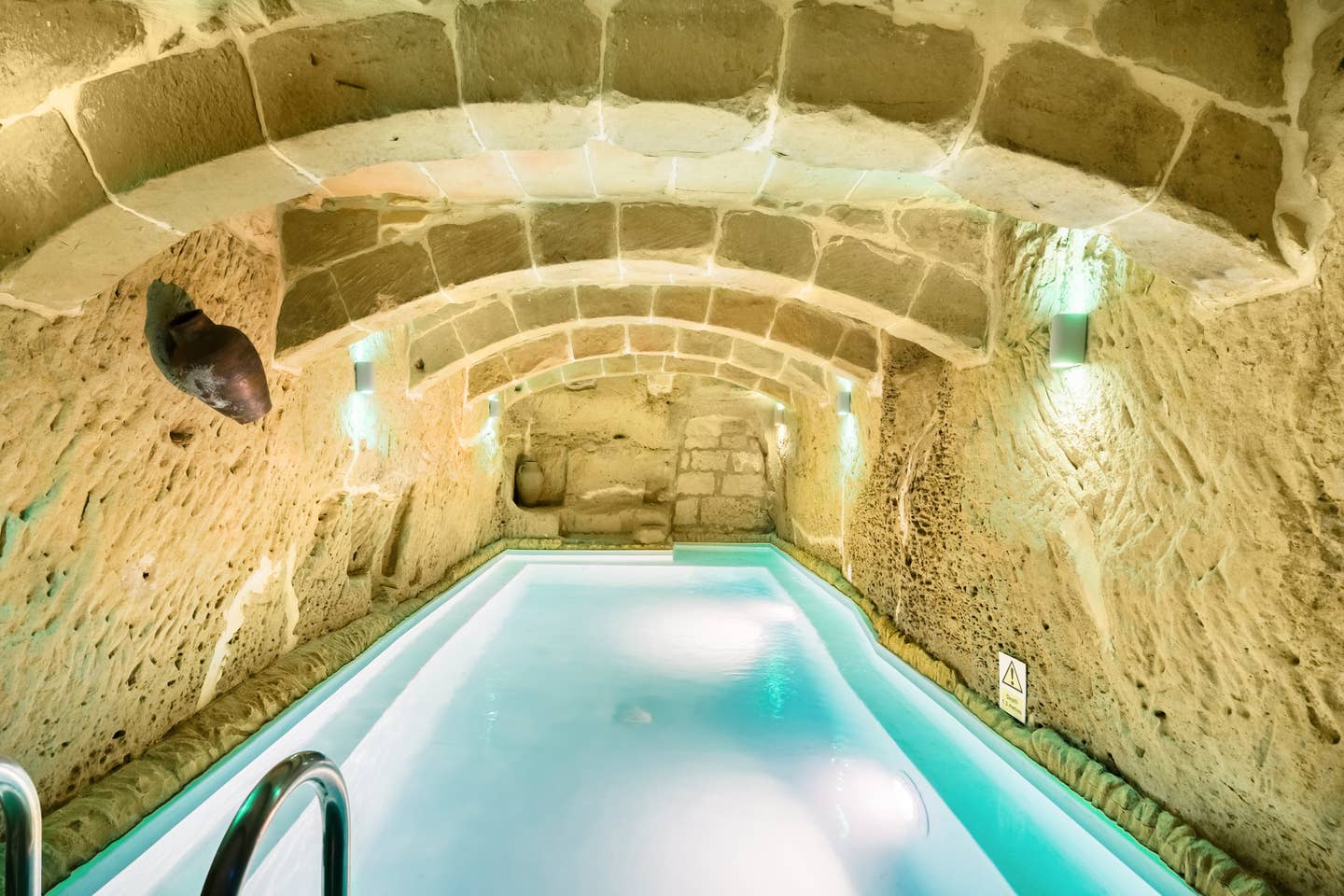The image depicts a unique indoor pool set within a rocky cave-like structure. The pool is long and narrow, with shimmering blue water reaching right up to the edge. On the left side, the upper portion of a silver ladder descends into the water. The structure surrounds this pool with walls in a tan, textured stone, giving a cave-like impression. Above the pool, cinder blocks or bricks, held together by white mortar, form arches that support the ceiling. Rows of these stone blocks stretch overhead, creating a rugged yet structured appearance. The ceiling also features white light fixtures, which emit light from both the top and bottom. Underwater, on the right side, two additional lights can be seen glowing beneath the surface. This ambient lighting further enhances the pool's tranquil and surreal atmosphere.